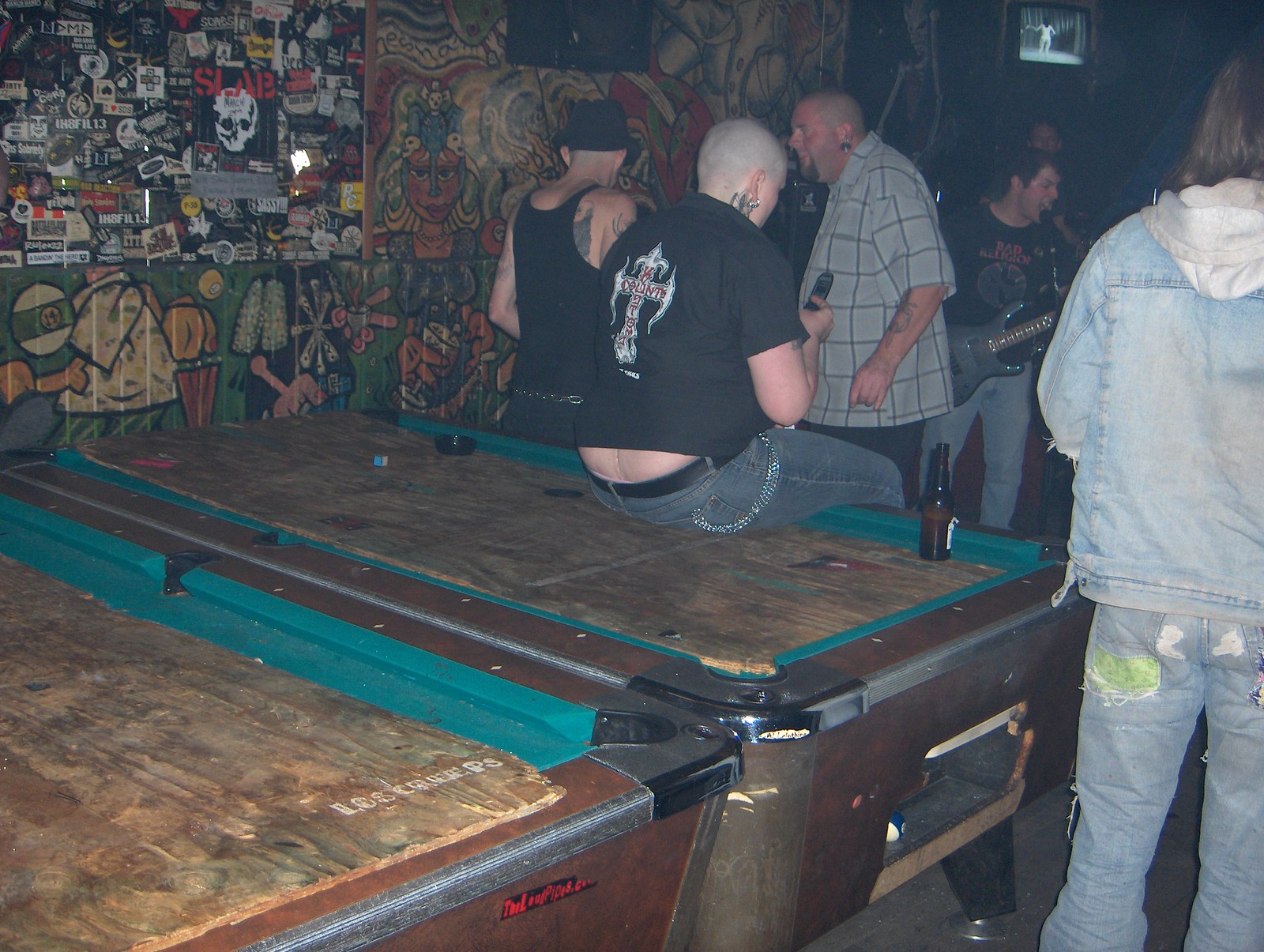This color photograph, set in a dimly lit tattoo parlor or a similarly dark establishment, possibly a bar, reveals a scene bustling with character and detail. Dominating the foreground are two horizontally aligned, worn wooden pool tables situated in the lower left. On the wall to the left, a vibrant collage of graphic images, including paintings and murals, some depicting white skulls and cartoonish figures, adds a layer of intrigue to the setting.

In the middle ground, five men, predominantly dressed in denim and black tops, are captured. Central to the scene is a bald man in a black tank top, flaunting tattoos on his right arm. Adjacent to him is another bald man in a black t-shirt adorned with a gold emblem on its back. To his right, a bald man in a black t-shirt with a cross on the back stands out. On the extreme right, another figure in a denim jacket and jeans, with their back to the camera, adds to the rugged ambiance.

Additionally, a musician is visible in the upper right section, gripping a guitar and singing into a microphone while donning a black t-shirt, further enriching the dynamic atmosphere of this intriguing location.